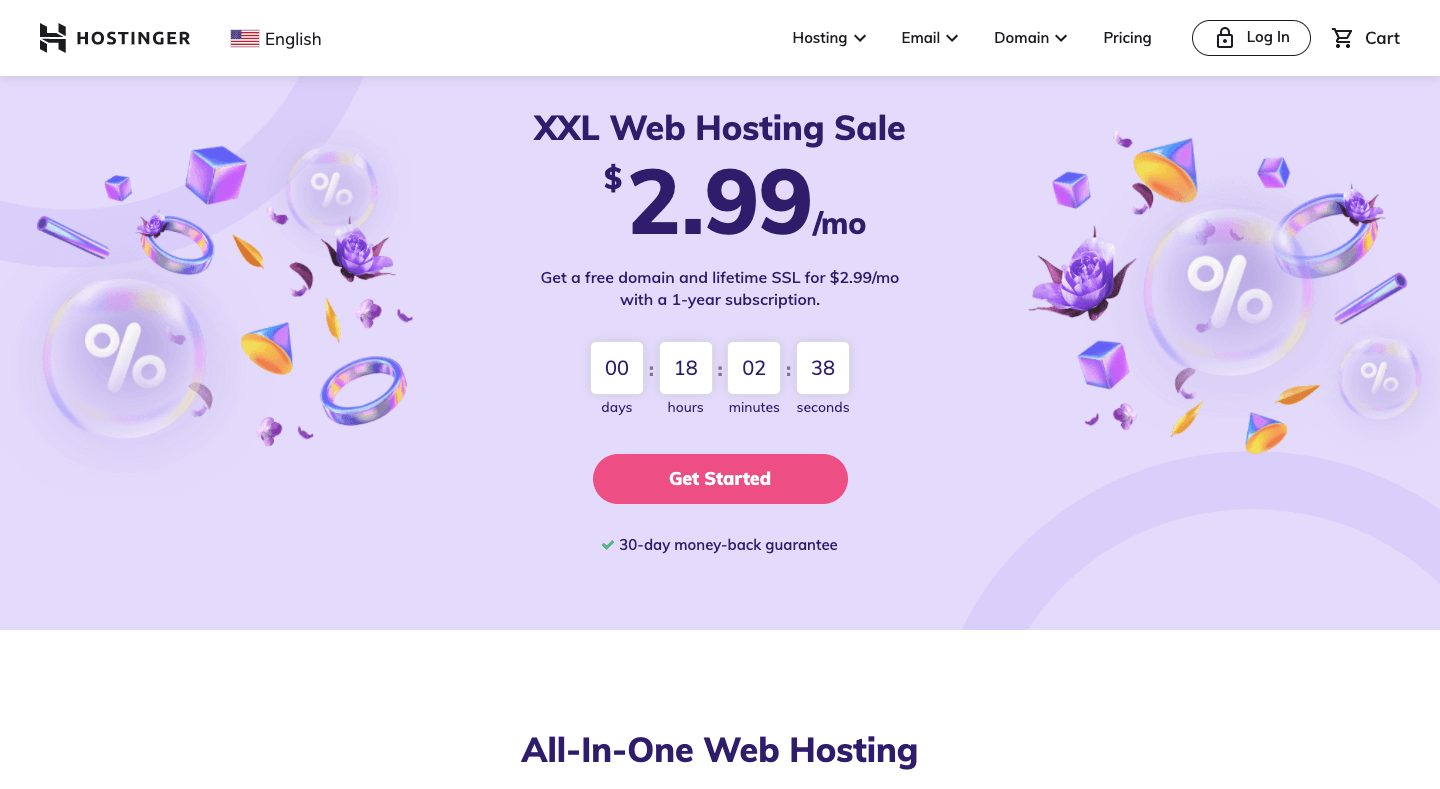The image displays a lavender-colored banner for Hostinger, spelled H-O-S-T-I-N-G-E-R, with the selected language set to English. To the right of the language setting, there is a menu in black text on a white background, offering options including Hosting, Email, Domain, and Pricing. Further to the right, there is an option for Secure Login and a shopping cart icon accompanied by the text "Cart."

The lavender banner prominently features the title "XXL Web Hosting Sale" in large, bold dark purple text. Below the title, it states in smaller text that users can get a free domain and lifetime SSL for $2.99 per month with a one-year subscription. There is a countdown timer beneath this information showing "0 days, 18 hours, 2 minutes, and 38 seconds" left for the sale. At the bottom of the banner, there's a striking pink button with white text that reads "Get Started."